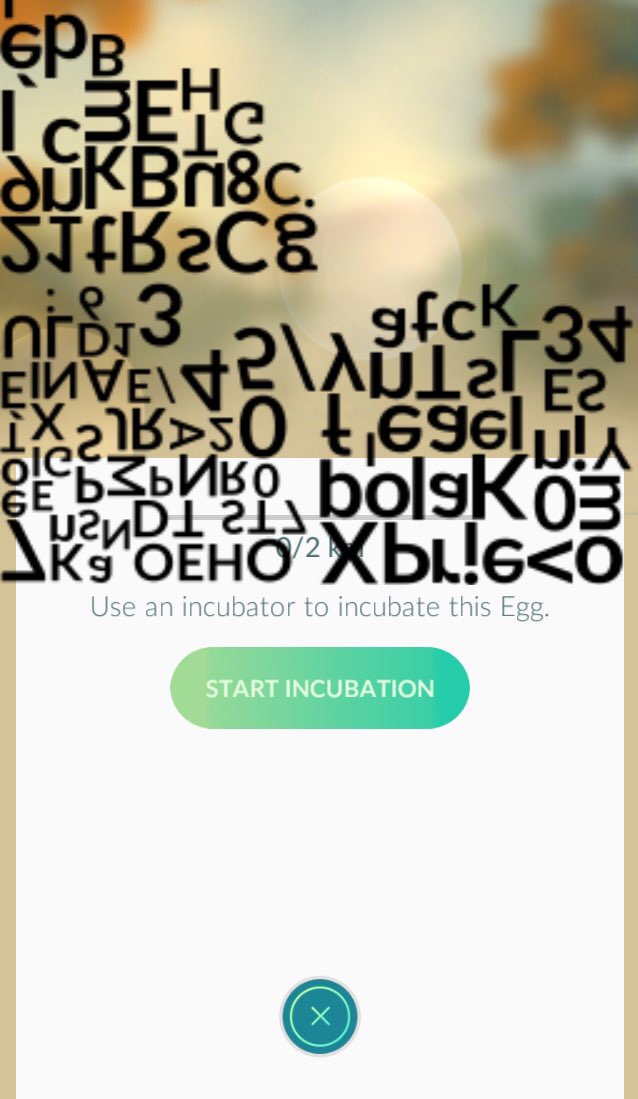The image appears to be a screenshot of a mobile app. At the top of the screen, there is a hazy, blurry depiction that could be a sun setting or rising behind trees, with muted colors including ochres, yellows, greens, and rust hues. This background may resemble an egg shape, fitting with the app's theme. Below this image, there are several alphanumeric symbols and letters, haphazardly arranged, some upside-down and sideways, resembling gibberish. Midway down the screen, a clear instruction reads, "Use an incubator to incubate this egg." Directly below this, there's a green, oval-shaped button with white text that says "Start Incubation." At the very bottom, a teal blue circle contains an 'X' for canceling the action. The purpose or exact nature of the app is unclear from the image provided.